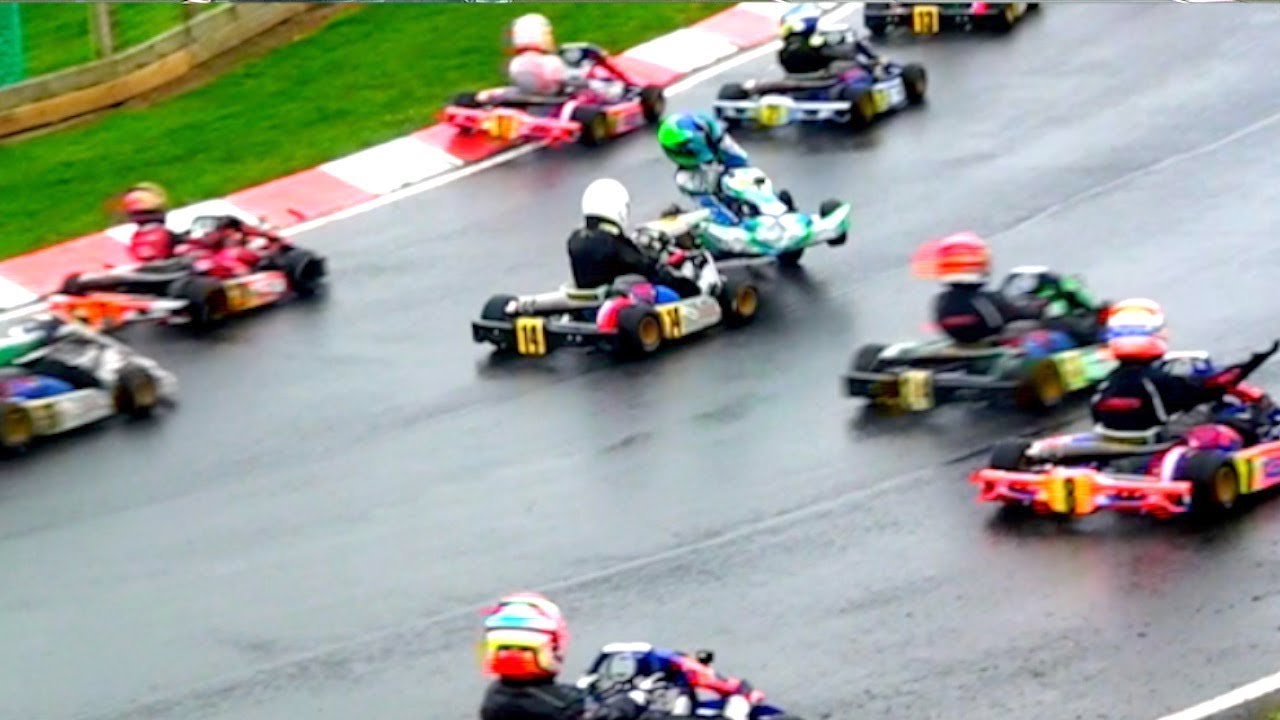The image captures an exciting outdoor daytime go-kart racing event on a wet, curving racetrack. The paved track, which is gray with red and white alternating border blocks, winds from the lower left to the upper right of the frame, broadening at the lower right corner. Nine competitors in brightly colored go-karts, ranging from red, blue, black, to white, can be seen zooming across the track, which appears wet along with the vibrant green grass on the left. Each driver, some of whom are little kids, is clad in a distinctive helmet-coloured and protective suit, speeding low to the ground. The photo also highlights the dynamic thrill of racing, with most go-karts appearing blurry due to their fast motion. In the top center, a notable moment is captured where one go-kart has collided with another, sending one spinning and partially up onto the other.